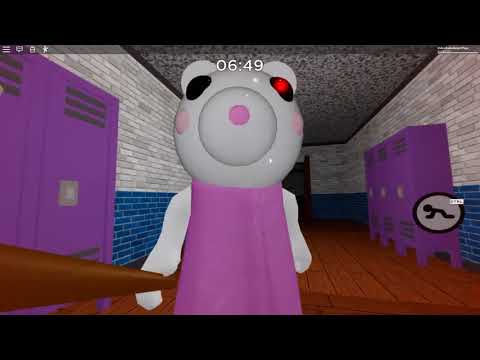This image is a pixelated still from a video game, reminiscent of a high school setting with a Minecraft-like style. In the background, you observe block-like walls; the upper half is white brick, and the lower half is blue brick. The floors are dark brown wooden planks. On either side of the hallway, there are vibrant pink lockers. A character stands prominently in the center, resembling a white bear with a round face and snout. The bear has black eyes, the right eye featuring a red dot. It is dressed in a pink or pinkish-purple dress and holds a bat in its left hand. Above the character, a countdown timer reads 06:49, and to the right, there's an icon of a stick figure doing push-ups, possibly indicating some in-game action or objective.